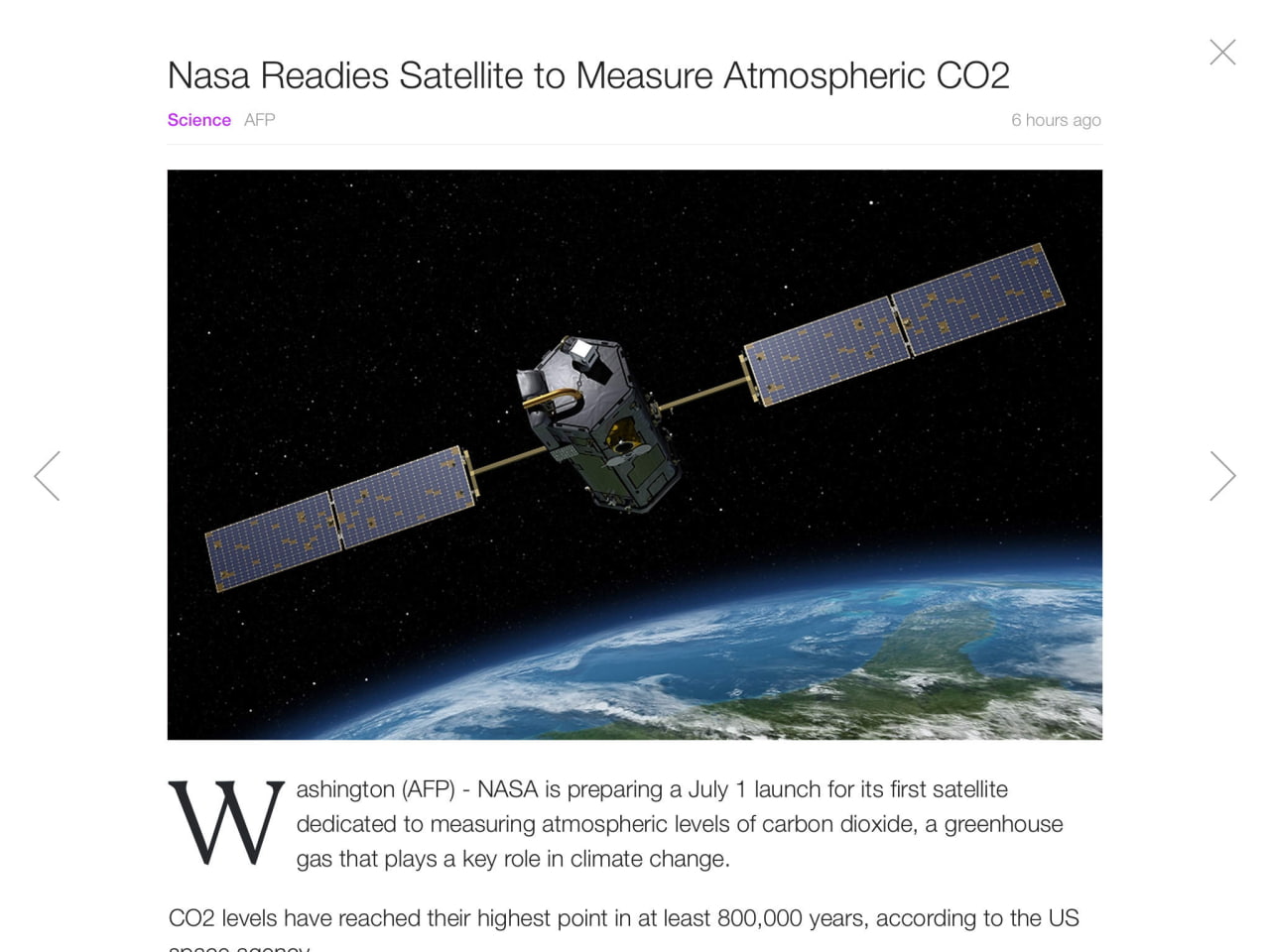In the image, a satellite equipped with four expansive solar panels, two on each side, floats gracefully against the vast backdrop of space. The satellite isn't a space shuttle, but a specific type of spacecraft designed for scientific observation. The inky blackness of space is dotted with twinkling stars, adding to the majesty of the scene. Below, the curvature of the Earth is visible, surrounded by a soft, ethereal hue. The planet's surface showcases sprawling oceans, swirling clouds, and intricate landscapes. This compelling photograph accompanies a news article from Washington, detailing NASA's preparation for a significant launch on July 1st. The launch, happening on the very day the image was captured, marks the deployment of the first satellite dedicated to measuring atmospheric levels of carbon dioxide, an essential step in understanding and combating climate change.